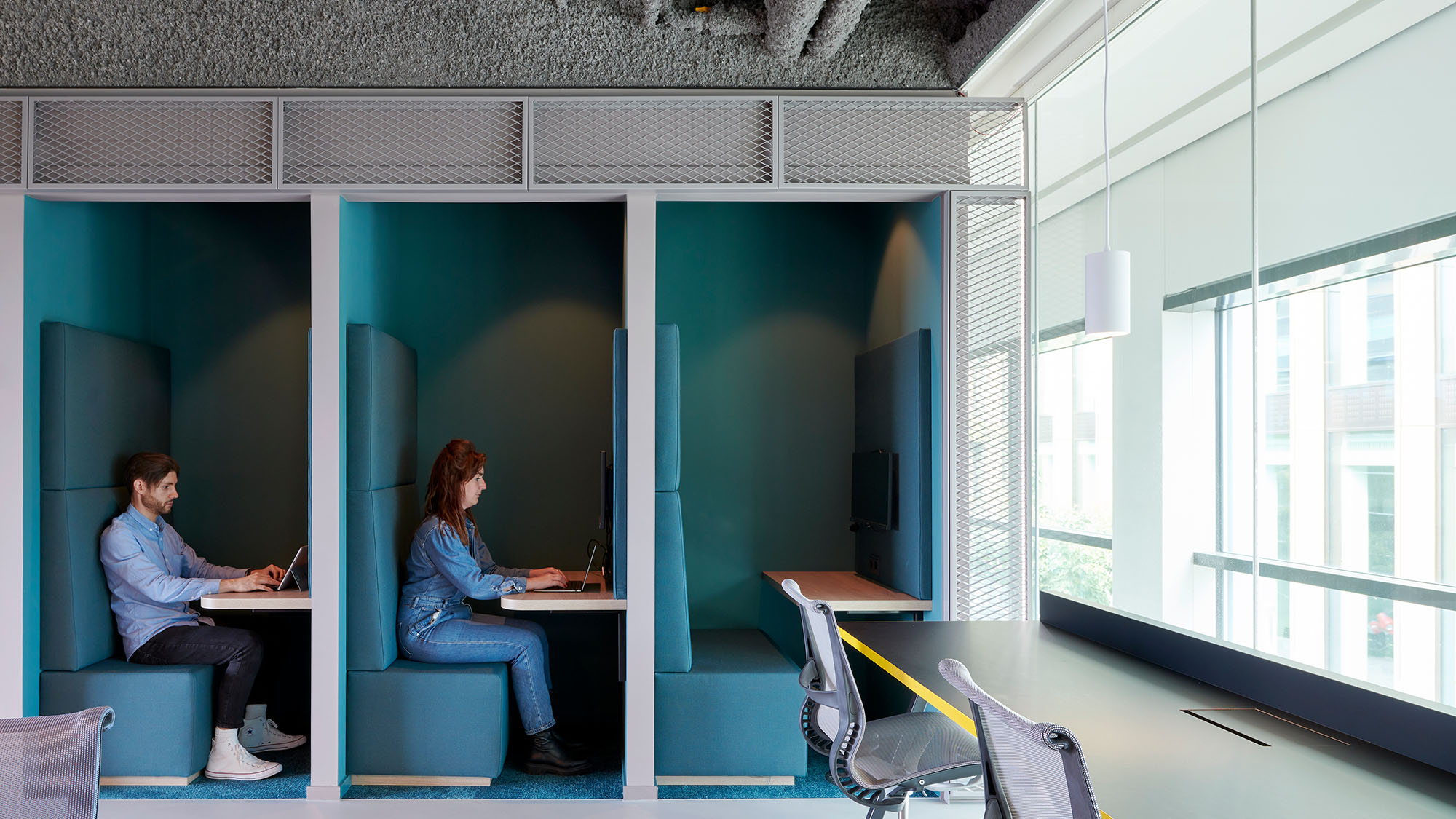The image depicts a brightly lit, indoor office setting with large windows on the right side, offering a view of adjacent buildings. In the foreground, at the bottom right, there is a desk. Adjacent to the windows, a counter with two computer chairs can be seen, oriented towards the windows. Perpendicular to this setup are three small, singular cubicles, each containing an upholstered bench and a small desk with what appear to be laptops or tablets equipped with keyboards. 

The leftmost cubicle is occupied by a younger man dressed in a light blue button-down shirt, dark jeans, white high-top sneakers, and sporting a light short beard. He is typing on his device. To his right, in the middle cubicle, a woman with medium-length brown hair sits typing on her tablet. She is dressed in blue denim jeans, black boots, and a matching jacket. The rightmost cubicle is empty. 

The space features white walls, drop-down lamps from the ceiling, and an open roof design that exposes the ventilation pipes. The entire scene has a computer-generated, realistic appearance, with human models that do not appear to be real.